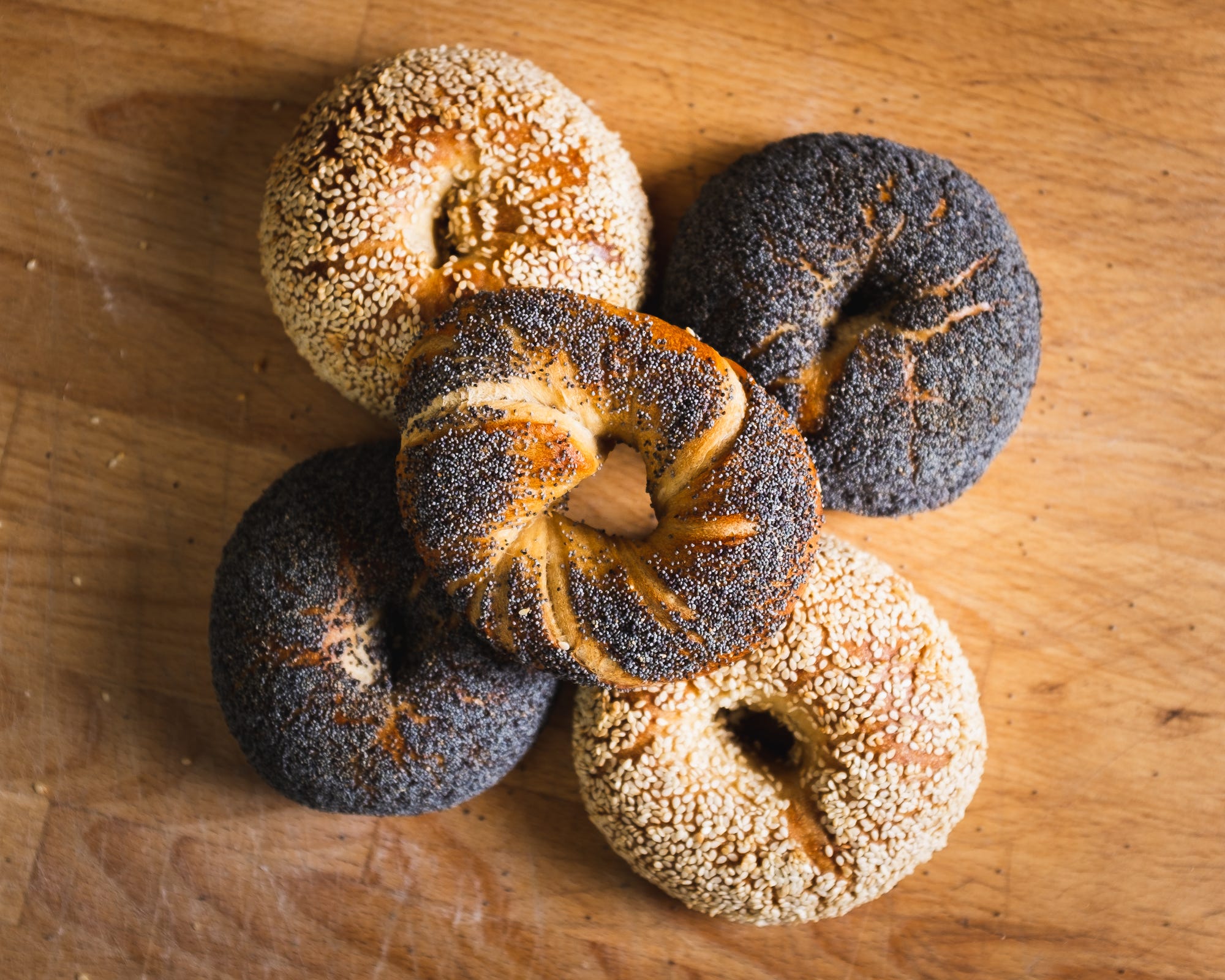This image features five bagels arranged on a worn wooden table that bears the marks of years of use, with visible knife scars and various blemishes. The bagels form a pattern with four laid flat and one positioned on top at the center. The bagels vary in appearance: two are coated in white sesame seeds, revealing only small patches of their rich golden-brown surfaces beneath the seeds, while three are adorned with nearly black poppy seeds. Among the poppy-seed bagels, two are densely sprinkled, and the third, positioned on top, is only partially covered, allowing more of its toasted brown surface to show through. The table around the bagels is scattered with some dropped seeds, both white and dark, adding to the rustic and well-used ambiance of a bakery workspace.